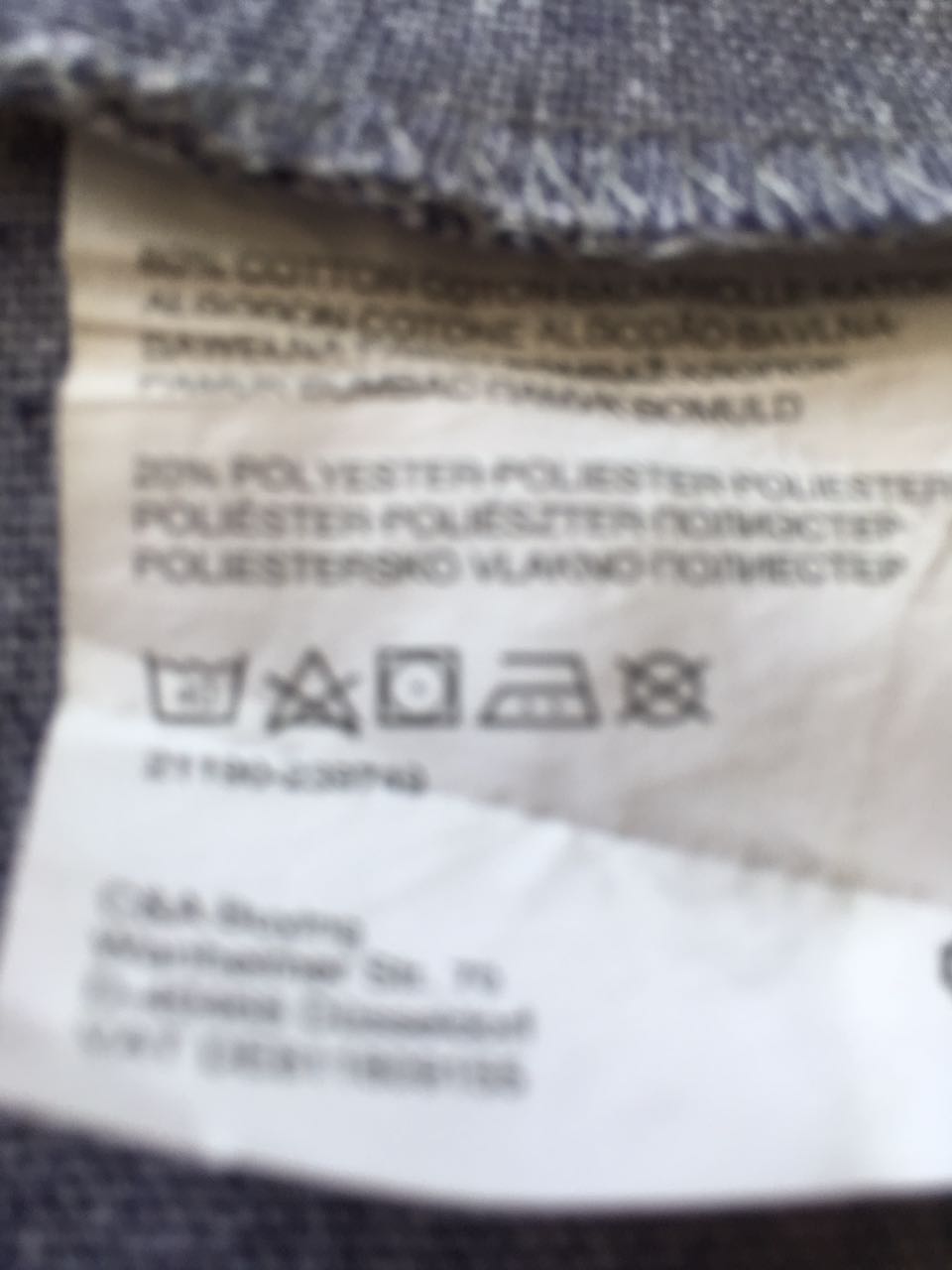The image features a white care label affixed to a piece of gray woven fabric which appears to be frayed and tattered at the top where the label is sewn. The white tag itself is slightly wrinkled with noticeable crease lines. It includes both text and symbols: the text lists materials such as cotton and polyester. The care symbols on the tag are: a washing machine, a triangle with an X through it, a square with a white circle in the center, an iron silhouette, a circle with an X through it, and additional text information underneath.